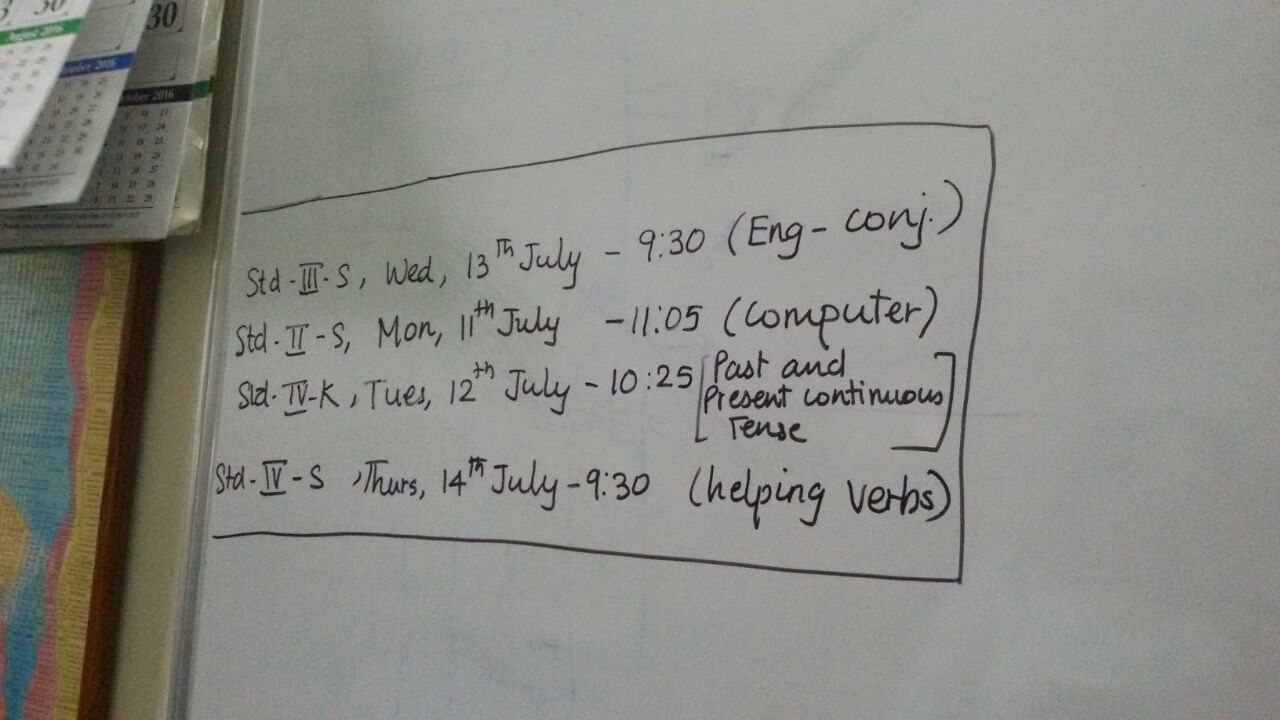The photograph depicts a classroom setting, focusing on the left side of a whiteboard. Drawn on the whiteboard is a long rectangular box containing the following scheduled information:
- "STD-3S, Wednesday, 13th July, 9.30, English Conjecture."
- "STD-2S, Monday, 11th July, 11.05, Computer."
- "STD-4K, Tuesday, 12th July, 10.25, Past and Present Continuous Tense."
- "STD-4S, Thursday, 14th July, 9.30, Helping Verbs."

In the upper left corner of the image, partially out of frame, there's a paper calendar barely visible, appearing to be pinned or hung up on the wall. The whiteboard and the detailed scheduling information dominate the right side of the image, while the wall and the calendar are seen on the left. The classroom scene suggests an organized plan for different lessons scheduled for various Standard (STD) classes throughout the week.